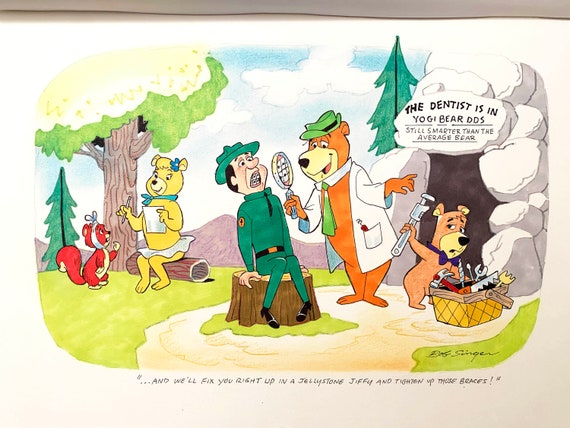In this hand-drawn illustration, possibly created with watercolors or colored pencils, we see a whimsical scene from the world of Yogi Bear. The focal point is Yogi Bear himself, clad in his iconic green hat and green tie, but this time he's donned a white medical coat and is holding a magnifying glass up to a park ranger's teeth. The park ranger, wearing a green uniform, sits on a stump leaning back, humorously displaying his teeth.

To the right of Yogi, Boo-Boo Bear, a smaller and lighter brown bear, is rummaging through a basket of tools, which include a hammer and a saw. He is handing Yogi a wrench, assisting in this makeshift dentist scenario. They are positioned in front of the entrance to a cave, above which a sign is chiseled into a rock, reading, "The dentist is in. Yogi Bear, DDS, still smarter than the average bear."

On the left side of the image, we see a female yellow bear sitting on a log, adorned in a white skirt with a green handkerchief and a blue flower in her hair. She interacts with a red squirrel that has a bandage or handkerchief tied around its head. The background features a blue sky with white clouds, a few trees, and additional greenery that give a playful, natural setting to the scene.

At the very bottom of the image, a caption reads, "We'll fix you right up in a Jellystone jiffy and tighten up those braces." This further adds to the comedic and lighthearted nature of the illustration, capturing the essence of Yogi Bear's charm.